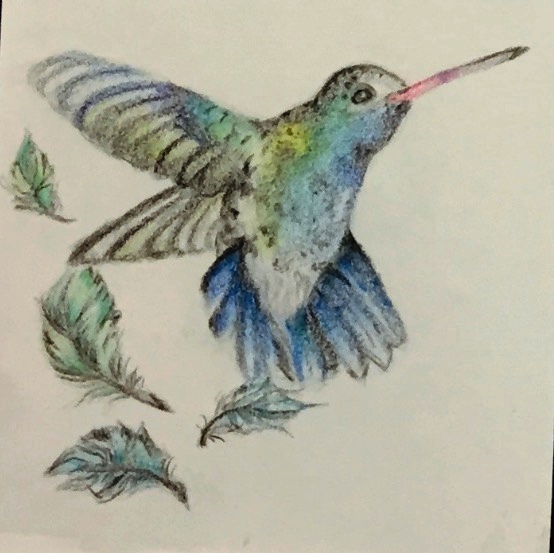This is a detailed drawing, likely created using pastels on white paper, of a hummingbird captured in mid-flight. The scene features the bird suspended in the air with its colorful wings flapping. The hummingbird's plumage is a striking blend of hues: its breast transitions from dark blue under its throat to pale blue, while its body showcases shades of blue, green, teal, yellow, and some gray. The bird's long beak is a gradient of pink closest to its head, fading to purple and finally a gray color. Its single visible eye is a gray color, adding a touch of realism to the image.

The wings of the hummingbird boast a greenish-yellow blend that transitions into varying shades of blue and cobalt, with the tips fading to a very light green or white. The tail feathers are predominantly cobalt blue with some white. The top of its head appears lightly colored, mainly white with a hint of blue shading. Adding depth and movement to the piece, feathers in greenish-blue and teal hues are depicted as having fallen off the bird or as floating softly behind, enhancing the sense of fluid motion and grace. The entire drawing is detailed with black outlines and definition that bring the hummingbird vividly to life against the backdrop of the white paper.